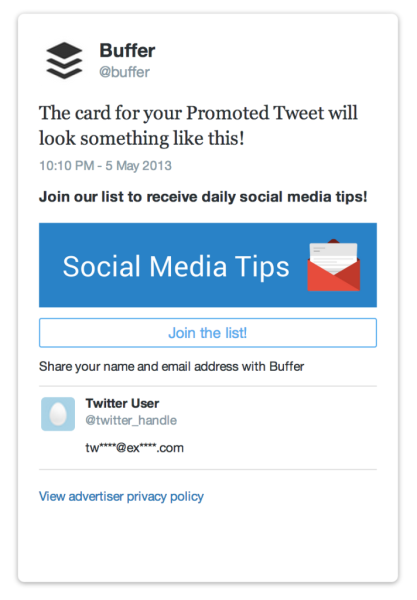In the upper left corner of the image, there are three black squares stacked vertically. To the right of these squares is the word "Buffer" written in black text. Below this, there's another line of text that says "@Buffer" in black. Further down, the text, "The card for your promoted Tweet will look something like this!" is displayed with an exclamation point, followed by a timestamp "10:10 PM - 5 May 2013."

Below this section, there’s a call-to-action message: "Join our list to receive daily social media tips!" which is punctuated with an exclamation point. Adjacent to it, within a blue rectangular box, the text "Social Media Tips" is written in white. To the right of this box, there is a red image of an envelope with a white piece of paper inside it.

Another informational section follows, stating "Join this list!" in blue text accompanied by an exclamation point. Beneath this, the text prompts users to "Share your name and email address with Buffer." Next to it, there is a small blue square containing an image of a white egg.

Finally, there's a line of text in black that reads "Twitter user @Twitter-handle," with the corresponding email, "tw at ex.com," below it. The last line of the image reads "View advertiser privacy policy" in blue text.